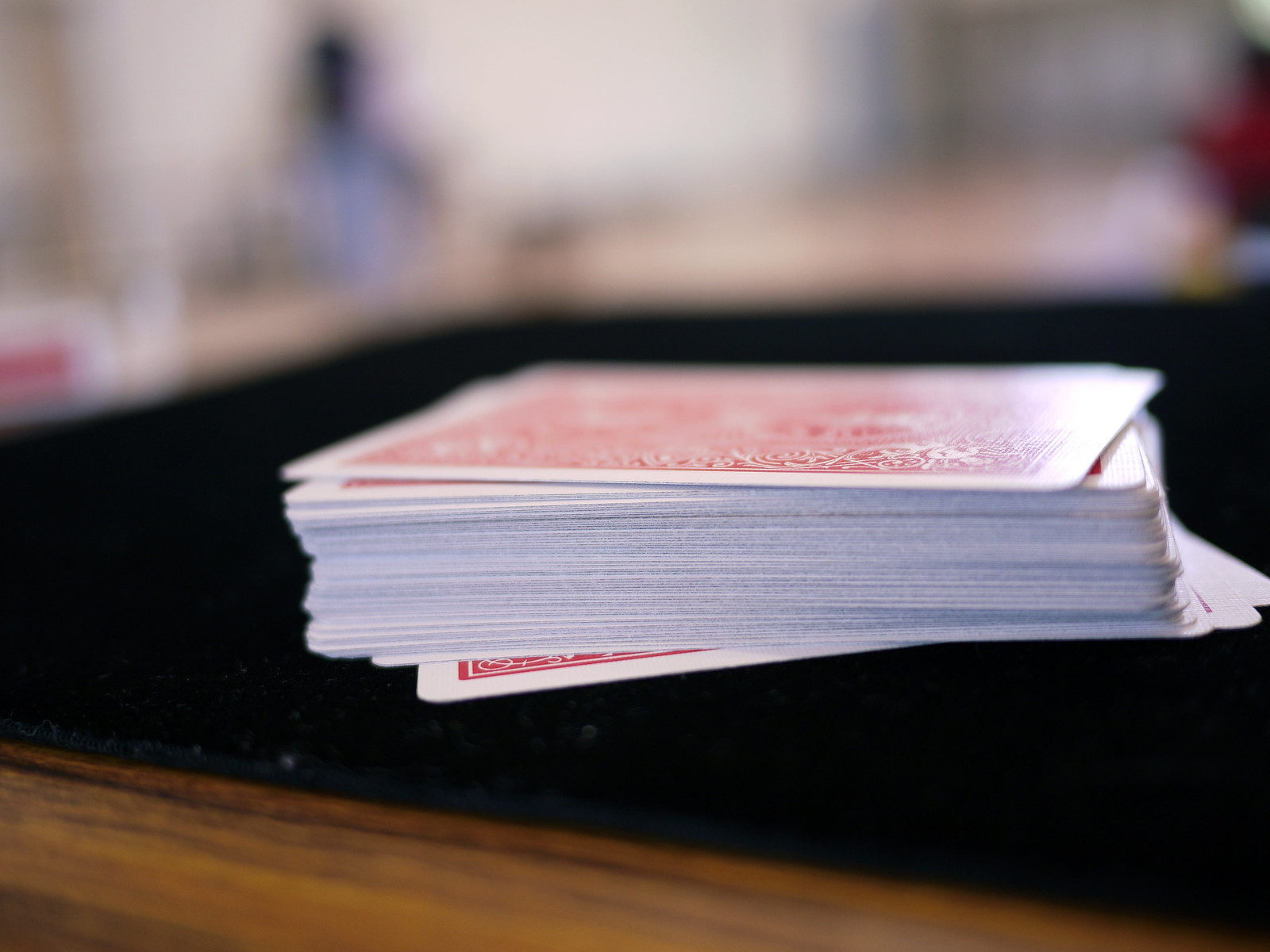The image captures a scene set against a light brown wooden table. In the bottom right corner, a stack of cards is prominently displayed. Each card features a white background with a red drawing, with the top card slightly askew and the rest aligned but shifted slightly to the right. The cards rest on a black, square-shaped soft mat that appears to be a mouse pad, occupying an area that extends from the bottom of the image upwards to about 10% from the bottom. 

In the blurred top half of the image, the right side shows a person with fair skin and dark hair. They are wearing a red shirt and have their arm resting on the table. Moving to the left, another individual with darker skin is discernible, wearing a lighter-colored shirt that appears bluish-white. In the top left corner, there is a rectangular, white and red reflective object, possibly a mirror, that seems to echo the colors of the cards below. The overall composition hints at a casual setting, perhaps a game night or a relaxed gathering.